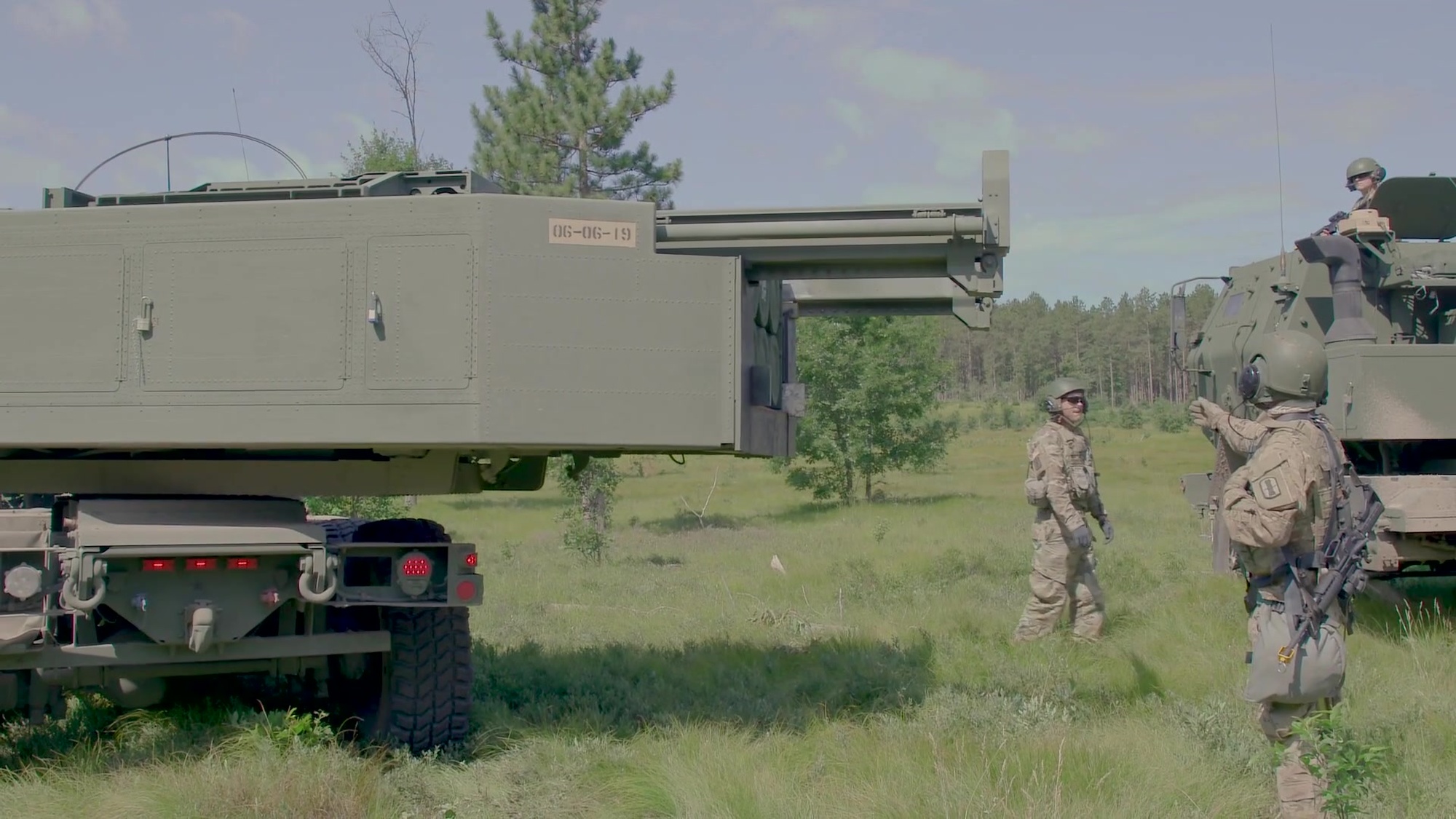The photograph, taken outdoors on a mostly clear yet faded day, captures a militarized scene featuring multiple vehicles and soldiers amidst a natural setting. The image, devoid of a distinctive border, is horizontally rectangular. At the top, the sky with scattered fluffy clouds forms the background, punctuated by a few pine and leafless trees. 

In the foreground, the left side showcases a modified Humvee, equipped with a swiveling piece of equipment that features metal latches, a rectangular device labeled "06-06-19", and what appears to be an antenna held by strings. To the right of it is another military-style vehicle, possibly a tank, partially obscured by the soldiers. 

Three soldiers, dressed in green fatigues and helmets, stand in the grassy field, their backs adorned with weaponry. One soldier is atop the armored vehicle on the right, adding a dynamic sense of activity to the image. The setting is densely wooded, with numerous trees and even barns visible in the background, lending a serene yet tense juxtaposition to the scene that hints at either a preparation for or practice of warfare.